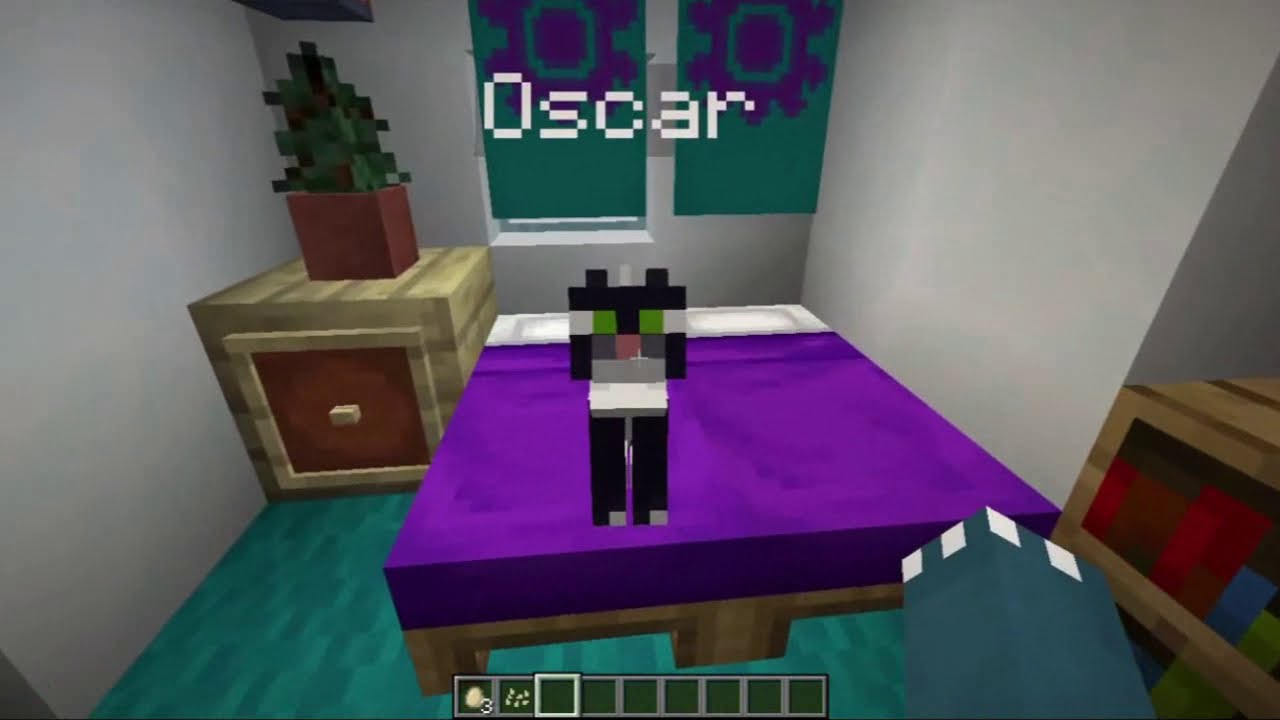This image appears to be a screenshot from the video game Minecraft, showcasing a blocky, 8-bit styled room, likely a bedroom. In the foreground, the player holds a dark teal-blue block with white checkers. Central to the image is a square, wooden bed frame topped with a purple bedspread and a white area, possibly representing pillows. Perched on the bed is a black and white pet with the name "Oscar" displayed above it. Oscar, which might be a dog or a cat, is sitting, showing its two black legs. To the left of the bed is a wooden nightstand with a small potted plant. The floor is covered in a turquoise or teal green carpet, and above the bed hangs a set of teal and purple curtains. The room's walls are entirely white, reinforcing the game's signature, cubic design.